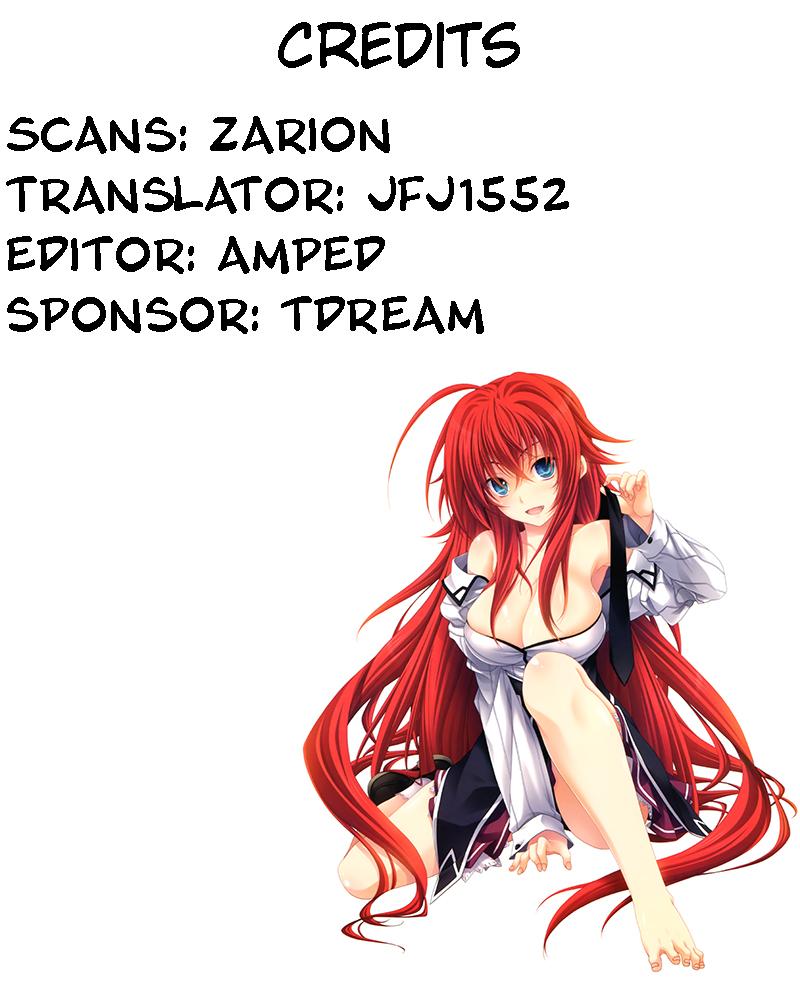The image depicts a popular anime character, likely from the series "High School DxD." She is a young woman with extremely long, swirling red hair that cascades down to her feet, layered and adorned with bangs. Her expressive big blue eyes and thin eyebrows add to her striking appearance. She is dressed in a silver off-the-shoulder dress that exposes her cleavage and features long sleeves, accentuating her figure, with an apparent nod to a school uniform aesthetic, particularly resembling a white shirt and a navy blouse. The girl is seated in a relaxed pose, with one knee bent and her other leg tucked behind her. Various credits such as "scans Z-A-R-I-O-N," "translator J-F-J-1-5-5-2," "editor A-M-P-E-D," and "sponsor T-D-R-E-A-M" are noted in the image, hinting at its artistic and collaborative creation process.